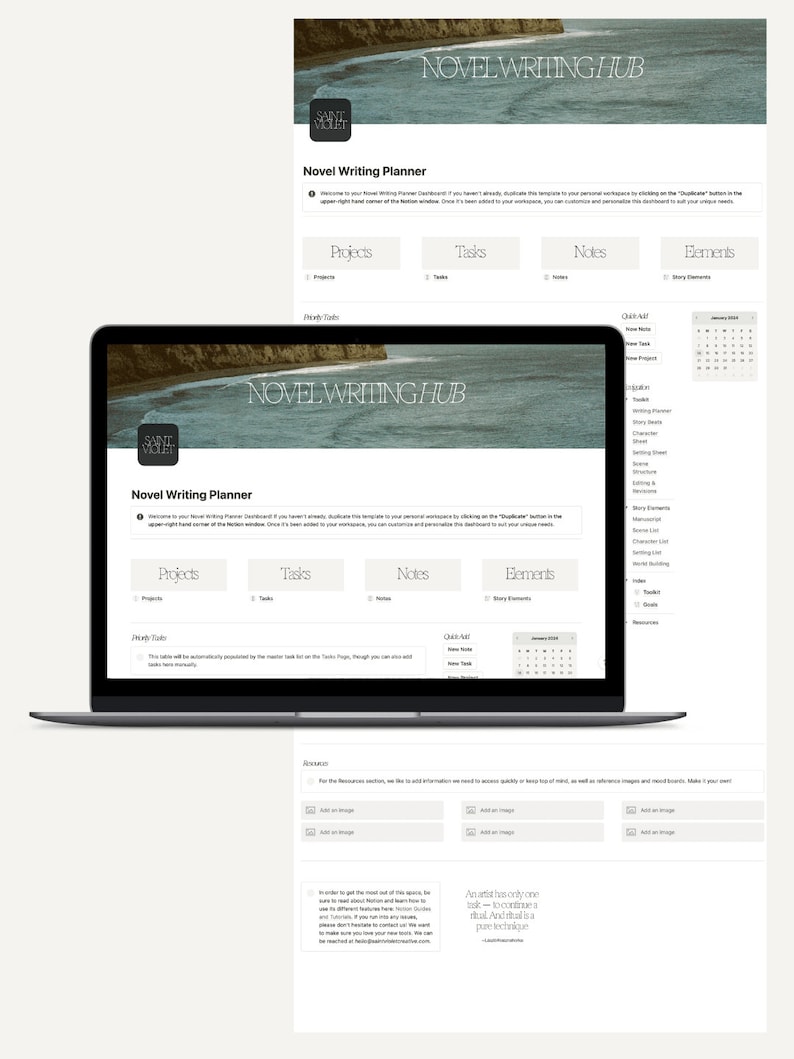Screenshot of the "Novel Writing Hub" webpage, designed to assist writers in completing their projects. The top banner features a serene nature scene depicting a coastline where waves crash against a cliffside, with a sandy beach nestled at its base. A small black icon is seen to the side of the banner. Below this, the main interface begins with a section titled "Novel Writing Planner," accompanied by a brief description. The interface includes four interactive buttons labeled: Projects, Tasks, Notes, and Elements. A compact calendar is positioned on one side, enabling users to track their progress over time. Centered within the screenshot is an image of a sleek, thin laptop featuring the same "Novel Writing Hub" screen on its display, characterized by a thin gray bottom and a black-trimmed bezel. Overlaying this, the background features additional layers of the "Novel Writing Hub" interface, creating an illustrative and visually cohesive presentation of the overall website's functionalities.